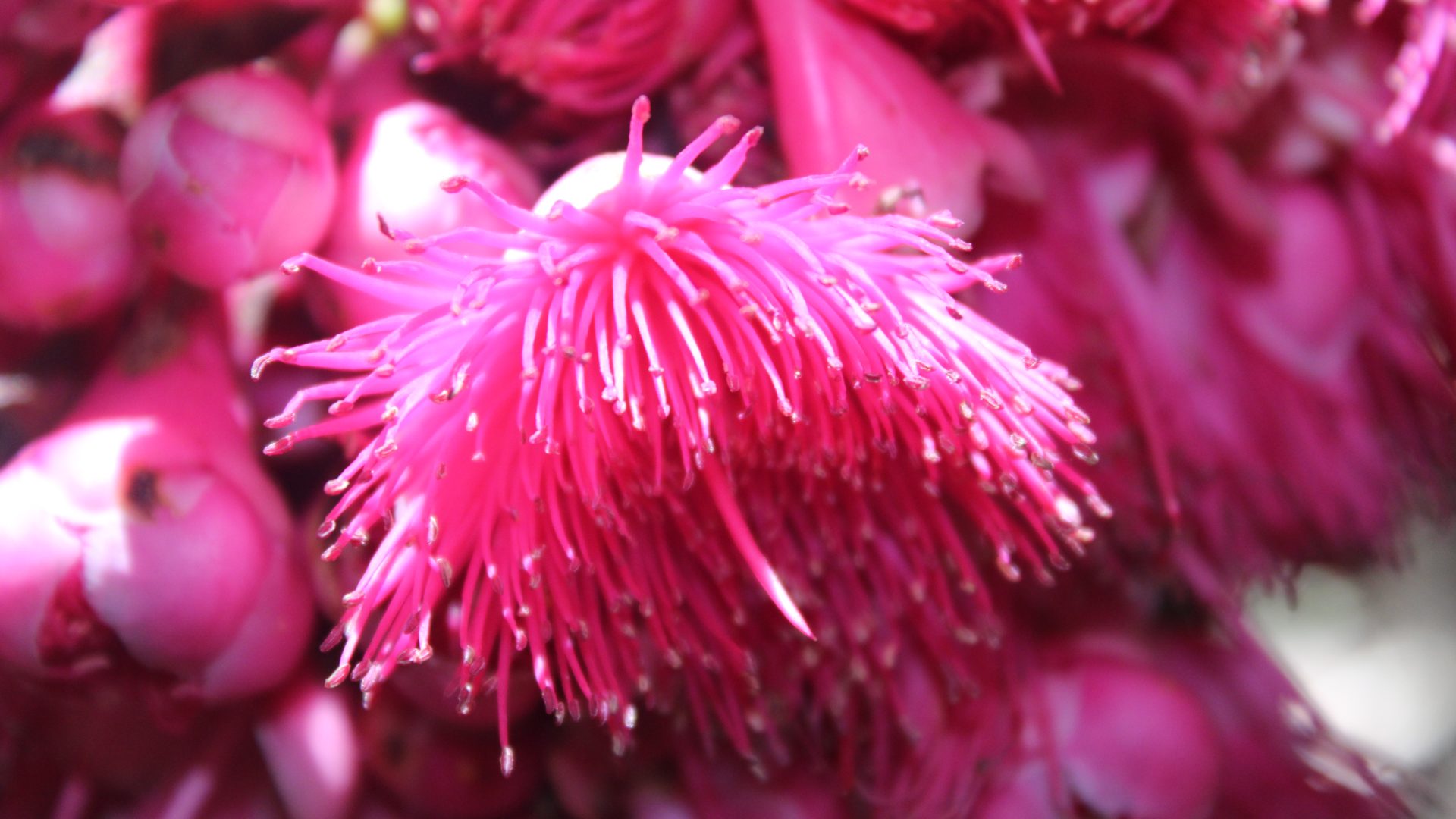The image features an ultra-close-up view of a vividly colored pink flower head with unusual tubular petals that droop towards the photographer. These tubular petals, which are predominantly pink with some white, create a striking visual effect reminiscent of tendrils or ruffled cheerleader pom-poms. In the blurred background, more flower heads with similar drooping tubular petals can be seen, adding to the sense of depth and focus on the central bloom. Additionally, the background also contains unopened bulbs or buds that resemble garlic or mini onion bulbs, contributing to the variety of shapes and textures. The setting is outdoors during daytime, as suggested by the natural lighting and absence of text or additional objects. The entire scene is dominated by various shades of pink, with occasional spots of brown, black, and off-white, enhancing the vibrant and dynamic nature of the photograph.